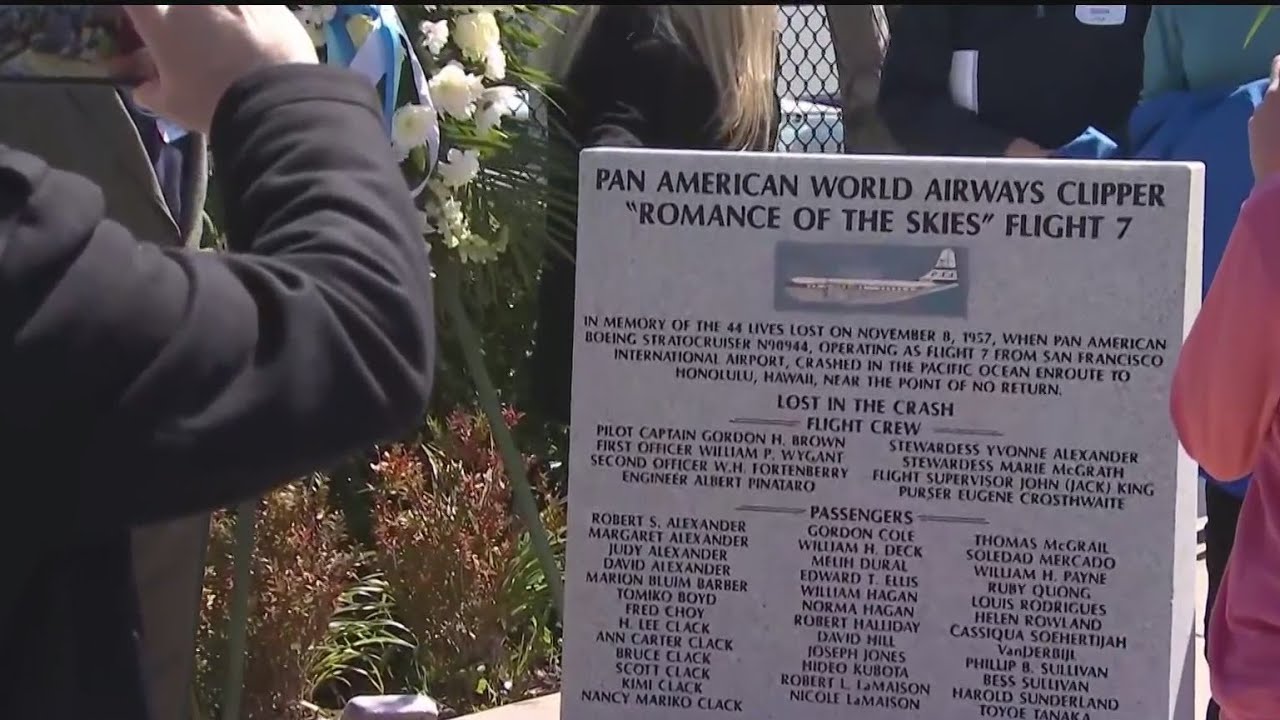The image is a rectangular outdoor photograph capturing a solemn ceremony. The focus is on a large, gray stone memorial plaque dedicated to the Pan American World Airways Clipper Romance of the Skies Flight 7. The plaque features a detailed tribute to the 44 lives lost on November 8, 1957, when the Pan American Boeing Stratocruiser N90944 crashed in the Pacific Ocean while en route from San Francisco International Airport to Honolulu, Hawaii. The memorial stone includes an image of the aircraft, the title of the flight, and lists the names of both the flight crew and passengers. Surrounding the memorial, people are gathered—visible from their torsos and dressed in formal black attire, suggesting the ceremony is in remembrance of the tragic event. To the left of the memorial, there is a large wreath adorned with white flowers and blue ribbons, emphasizing the commemorative nature of the gathering.